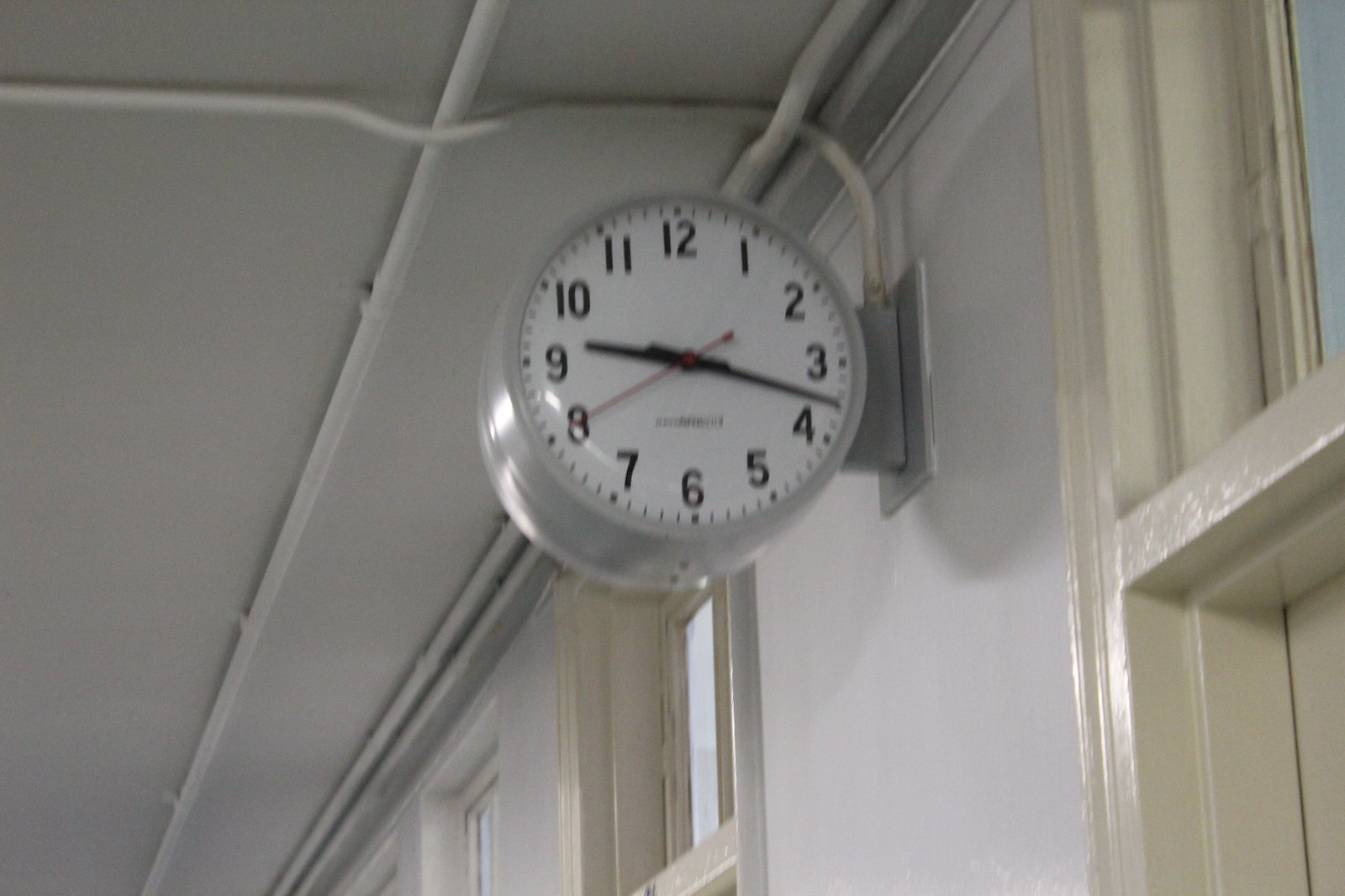The photograph showcases the interior of a building, captured from a vantage point directly below a prominently featured clock. The clock, which has a round, industrial design, stands out against the uniformly pale cream or white-painted surroundings. Suspended from the wall, the clock is mounted on the right-hand side by a sturdy block, with a metal conduit delivering power that extends upward from the block, continuing across the ceiling. The clock's face is minimalist, featuring a clean white background with black numerals in a straightforward typeface. The time displayed on the clock reads approximately 9:17. Below, the framing of doors is visible, further emphasizing the height from which the photograph is taken and the overall functionality of the space.